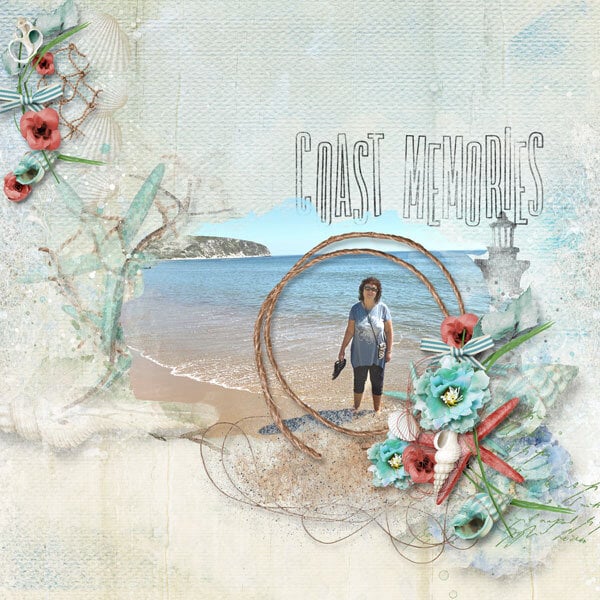The square image appears to be a scrapbook memory of a serene vacation, featuring textured backgrounds reminiscent of napkin material and an intricate design overlay of seashells, blue flowers, a sea star, and coral-colored flowers extending from the bottom right to the top left. Toward the left near the top, a plant stem tied with a white and blue striped bow paired with pink flowers adds to the decorative elements. Dominating the center of this collage is a rough-bordered photograph framed by a circular brown rope, slightly to the right of the image. The photo captures a smiling woman in her 40s with long brown hair and sunglasses. She is standing in the water on a sunny beach with her bare feet embraced by the shore's gentle waves and a distant cliff backdrop. The woman is dressed in capri pants, a long blue tunic featuring a white picture on the front, and a white bag draped across her chest to her hip. She is also holding a pair of black shoes. Just above this central photograph, the words "Coast Memories" are prominently displayed in black border font, with a lighthouse graphic subtly positioned to the right.